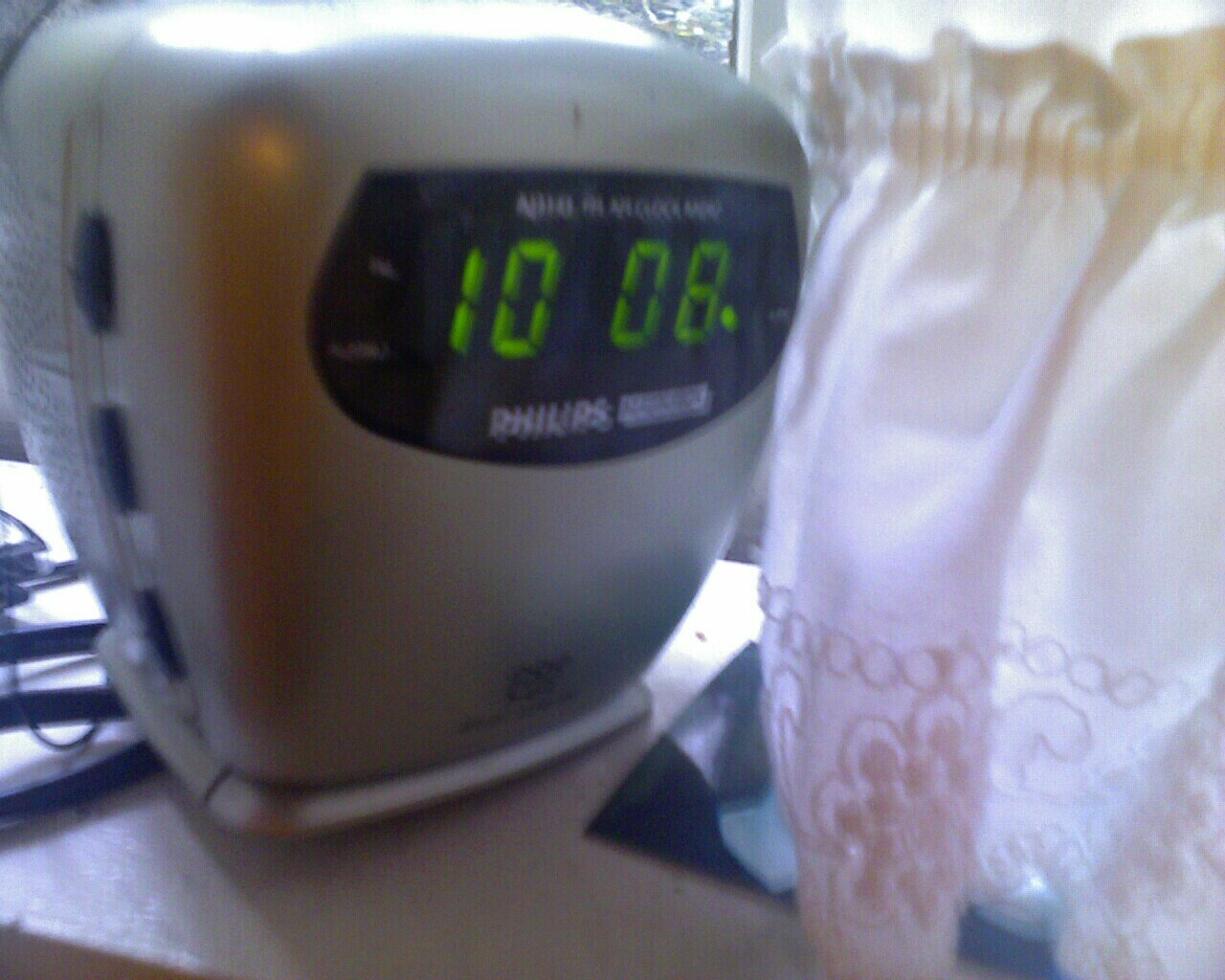The image depicts a slightly blurry, small gray Philips device with a rectangular black screen displaying green numbers "10:08." A green dot is visible to the right of the numbers, and three black rectangular buttons are located on the side of the device. The device is resting on a table, with some cords trailing behind it. To the right of the device, there's a white, crimped cloth or doily with a lace or floral design at the bottom. In the background, there is either a window or sliding glass door, with an outside view of bushes or a TV screen showing a nature scene.